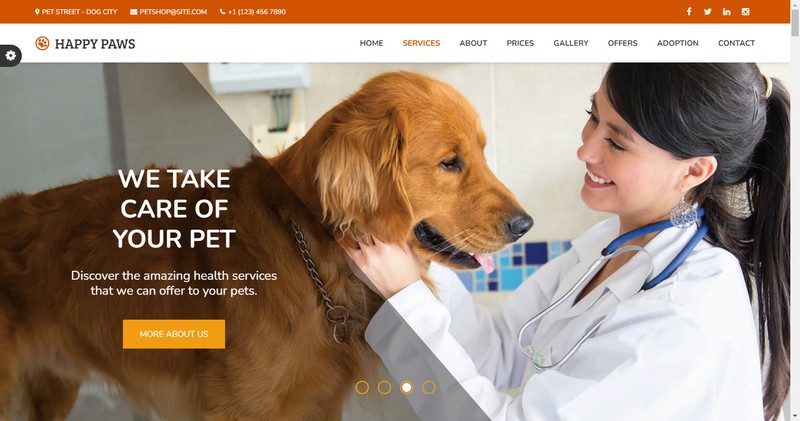The website "Happy Boss" prominently features a welcoming and professional image of a female veterinarian with long black hair tied in a ponytail, dressed in a white lab coat and stethoscope, providing an examination to a golden retriever standing on a table. On the dog's side, there is a caption in white lettering that reads, "We take care of your pet. Discover the amazing health services that we can offer your pets." Below the image is a yellow square button with white lettering that says, "More About Us."

In the top section of the website, the title "Happy Boss" is followed by a navigation menu with several options: Home, Services (highlighted in yellow indicating it is currently selected), About, Prices, Galleries, Adoptions, and Contact. The website also displays icons for their social media presence on Snapchat, Facebook, Twitter, and LinkedIn.

At the bottom of the image, four navigation bubbles are visible, with the third bubble filled in yellow, indicating that it is the third image in an auto-scrolling sequence. The page also contains advertisements for various pet-related services such as PetSmartDogCity, PetSmart, PetShop.Site.com, and includes a placeholder for a fake phone number. This detailed layout showcases "Happy Boss" as a comprehensive online destination for animal welfare information and services.